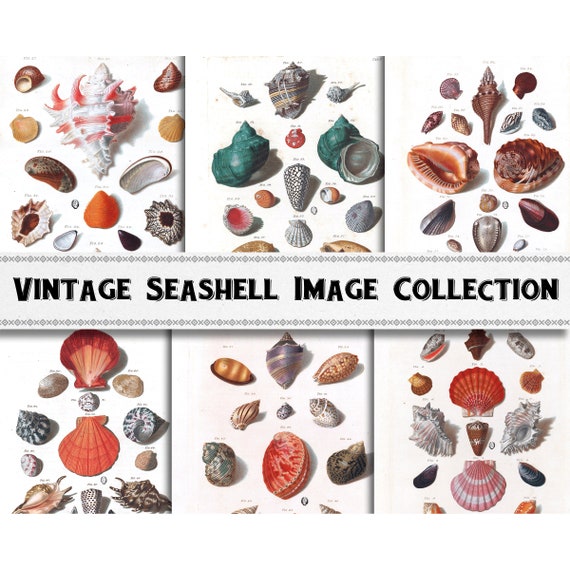The image is titled "Vintage Seashell Image Collection" and features a collage of six distinct grids, each showcasing a variety of seashells against a white background. The text labeling each shell is too small to read, but the diverse array of seashells can be described in detail. The collection includes shells of various sizes and shapes, such as conch shells with intricate whorls and spirals, smooth cylindrical shells, and classic clamshell shapes. The shells display a wide range of textures and colors, including black, white, gray, brown, off-white, red, teal, purple, and orange. Some shells are spiky, while others are smooth, and there appear to be pearls scattered among them. Each grid contains close to a dozen shells, highlighting the vast diversity within this vintage collection.